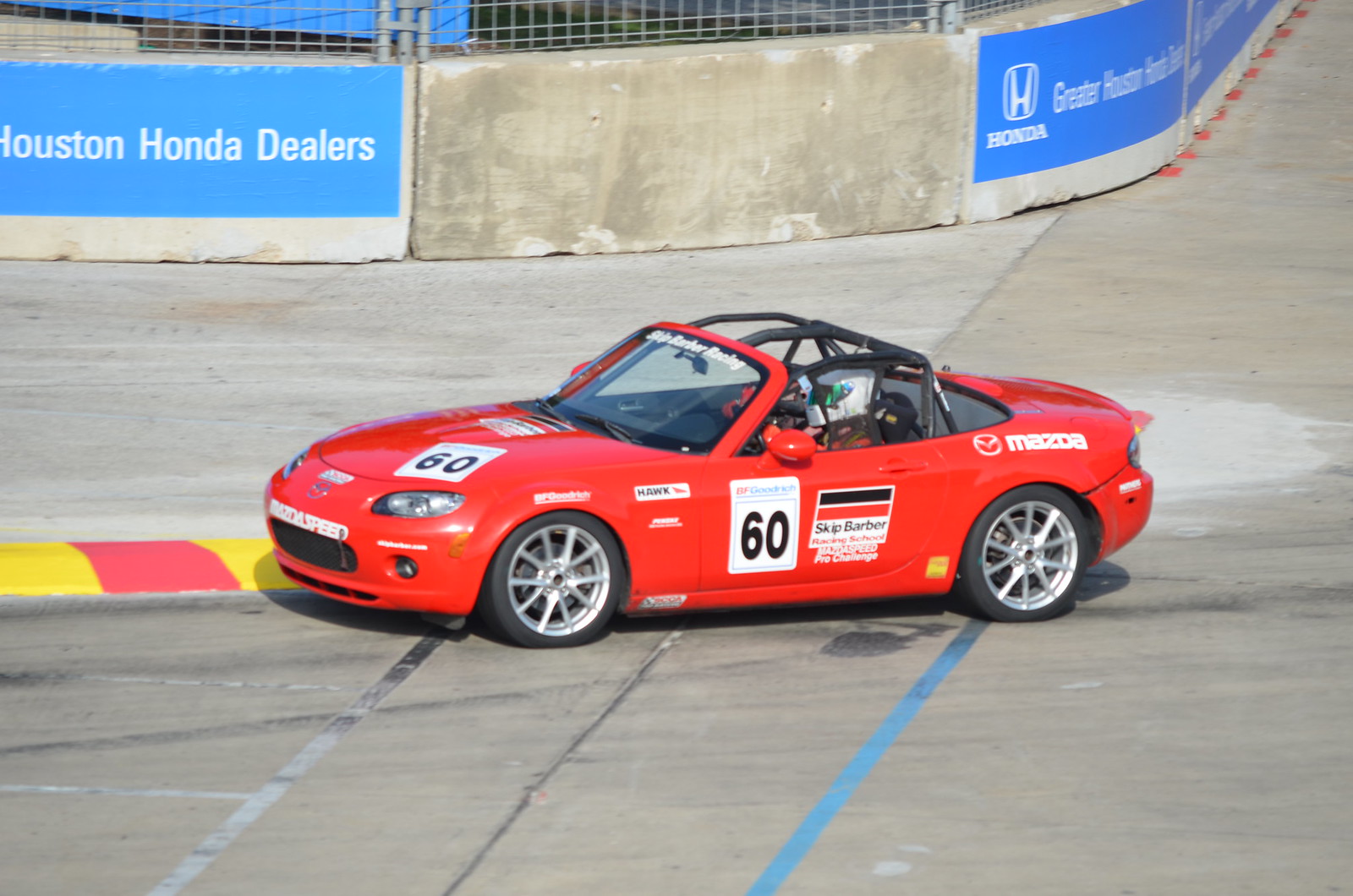This image features a bright red race car, prominently displaying the number 60 in black text on a white background, positioned on both the side and hood. The car, which is a convertible Mazda adorned with a variety of decals like Mazda and Skip Barber Racing, features silver rims and a robust roll cage. A driver, wearing a white helmet with green visors, sits in the car, which is in motion, navigating a turn to the left on a concrete racetrack. The track itself is bordered by concrete barriers and a stone wall, with advertisements for Houston Honda Dealers clearly visible on banners in the background. The windshield also sports a writing related to Skip Barber Racing. There are also distinct curb markings in a yellow and red pattern next to the car. The scene is captured in broad daylight, enhancing the vividness of the car and its surroundings.